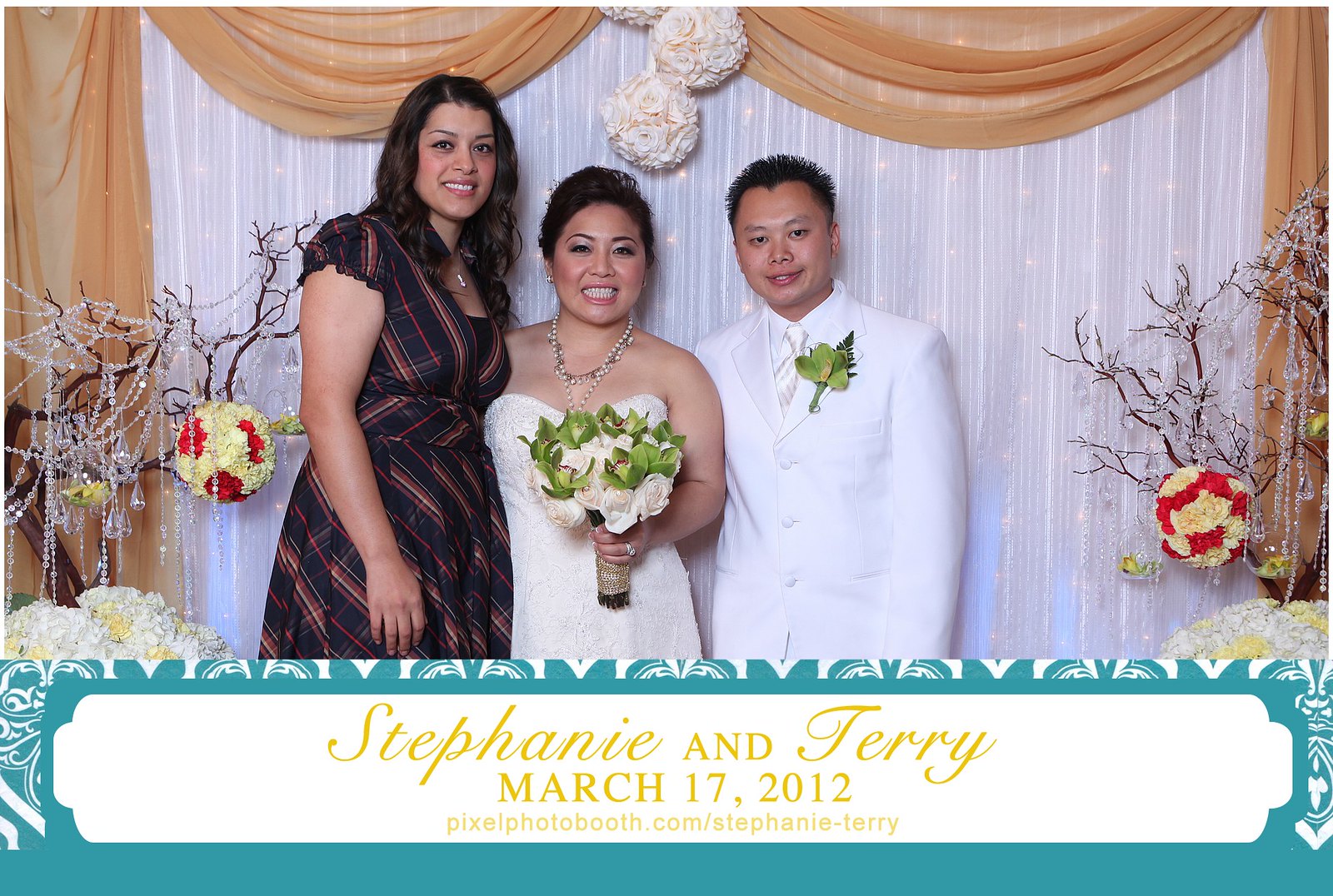This detailed color photo captures a wedding scene featuring three individuals set against a backdrop of ornate decorations. From left to right, there is a taller woman with shoulder-length dark hair and brown skin, likely of Hispanic descent, wearing a dark dress with red stripes and white lines. The bride stands in the middle, smiling in a sleeveless, strapless white gown with a sweetheart neckline. She holds a bouquet of white roses and wears a pearl necklace. To her right is the groom, clad in a full white tuxedo with a green corsage on his lapel. Both the bride and groom appear to be Asian. The background showcases an elaborate white curtain with a gold overhang, flanked by tree branches adorned with crystals and white, snow-like flowers. Below the image, a turquoise banner holds a white rectangle with gold script reading "Stephanie and Terry, March 17, 2012," followed by the text "pixelphotobooth.com/Stephanie-Terry."